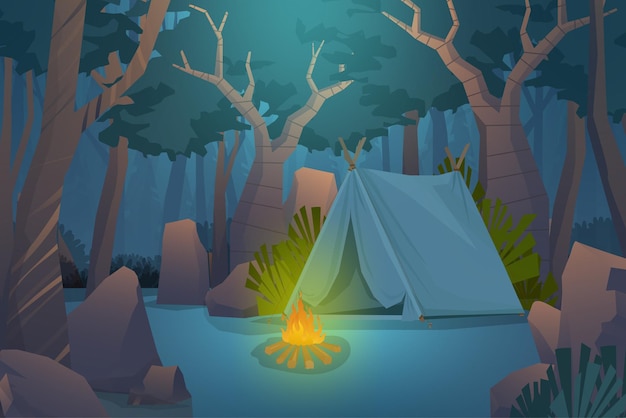In this cartoonish nighttime forest scene, the focal point is a white pitch tent with its front slightly open, draped partially covering the entrance. Positioned directly in front of the tent is a small campfire with vibrant orange flames surrounded by six fanned-out logs. The ground is depicted in dark teal hues, giving the impression of grass without detailed textures. Scattered around the campsite are protruding brown stones and large boulder-like rocks. The backdrop features tall brown trees with horizontal dark brown stripes along their trunks, extending upward and branching off near the top. The upper third of the image is filled with lighter and darker green foliage, adding depth to the dense forest setting. The campfire's glow softly illuminates the surrounding green leaves and bushes, enhancing the sense of a cozy, secluded spot in the wild.